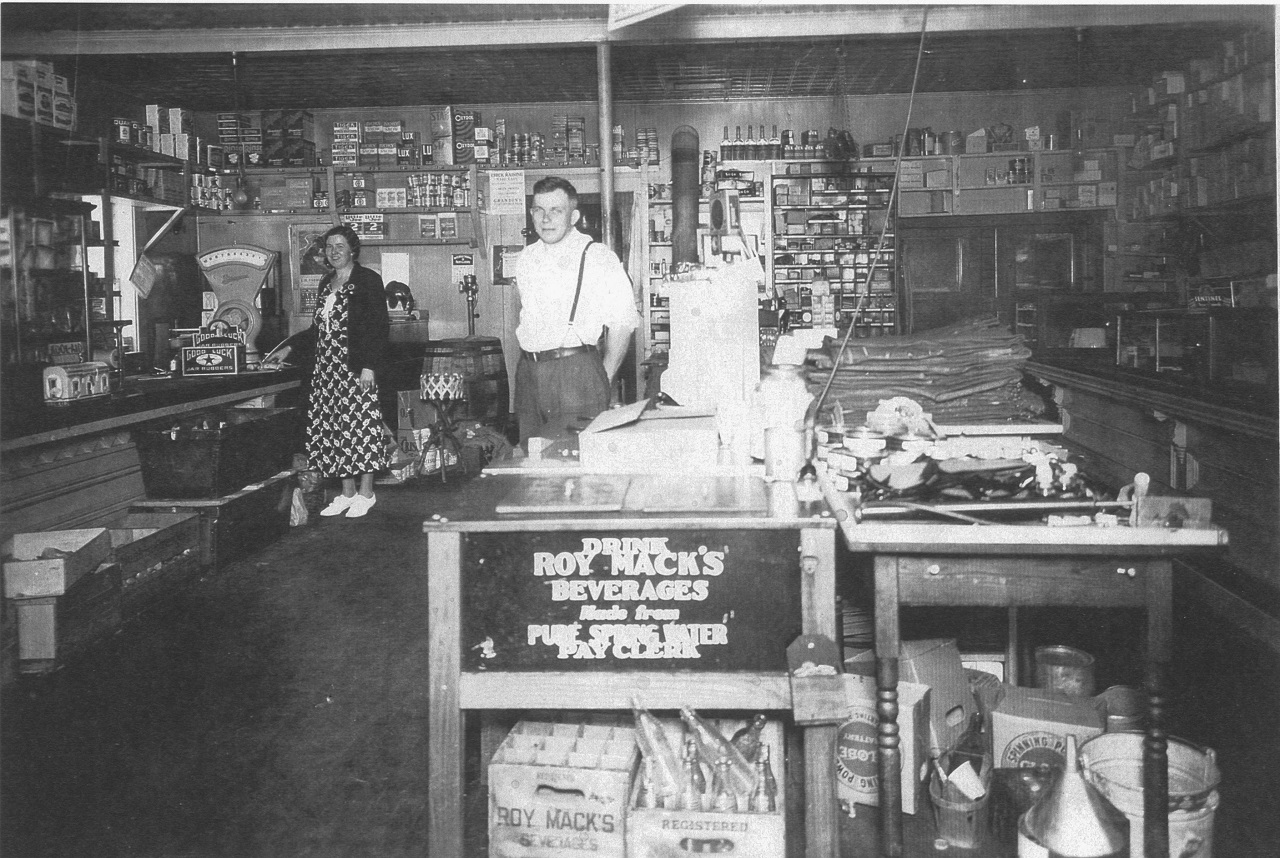This black and white photorealistic image captures the interior of an old general store, likely from the 1930s or 1940s. The foreground prominently features a sign advertising "Roy Maxx beverages made from pure spring water, pay clerk," accompanied by a case of glass bottles arranged in wooden boxes with bottle separators underneath. The store is stocked with a variety of goods typical for the era, including tools, hardware, a scale, and possibly buttons and ribbons. The walls are densely lined with various items. A man in a white shirt, jeans, and suspenders stands near a pole, gazing directly at the camera. In the background, a woman dressed in a checked dress, white sneakers, and a black sweater smiles towards the lens, positioned farther back at the counter. Presumably, these are the proprietors of the store. The overall impression is one of a bustling, well-stocked mercantile establishment, offering a glimpse into a bygone era.